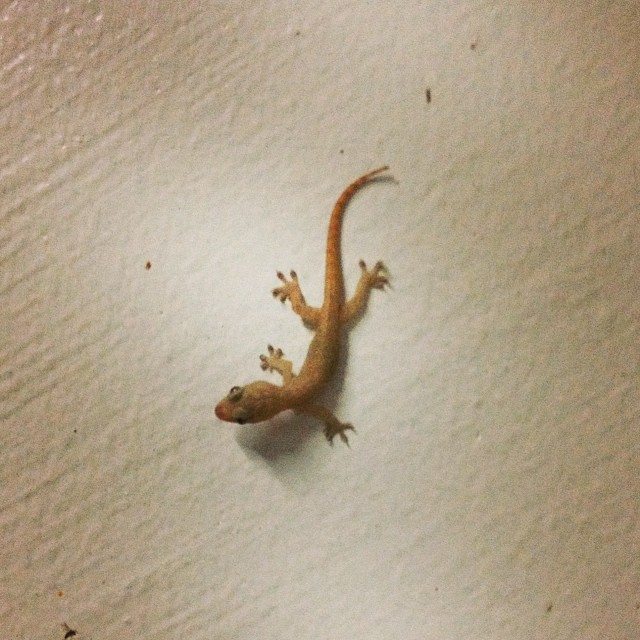The image depicts a small gecko hanging upside down on a slightly textured white wall with subtle stripes going towards the left. The light tan lizard, featuring black protruding eyes and pads on its toes, is situated right in the center of the photograph. Its tail, which transitions to a richer orange-tan color, points towards the right side of the image while its head is turned towards the left. The gecko, appearing slender and only a few inches long, is staring leftwards. Additionally, there is a tiny grey fly or insect visible at the bottom of the image.